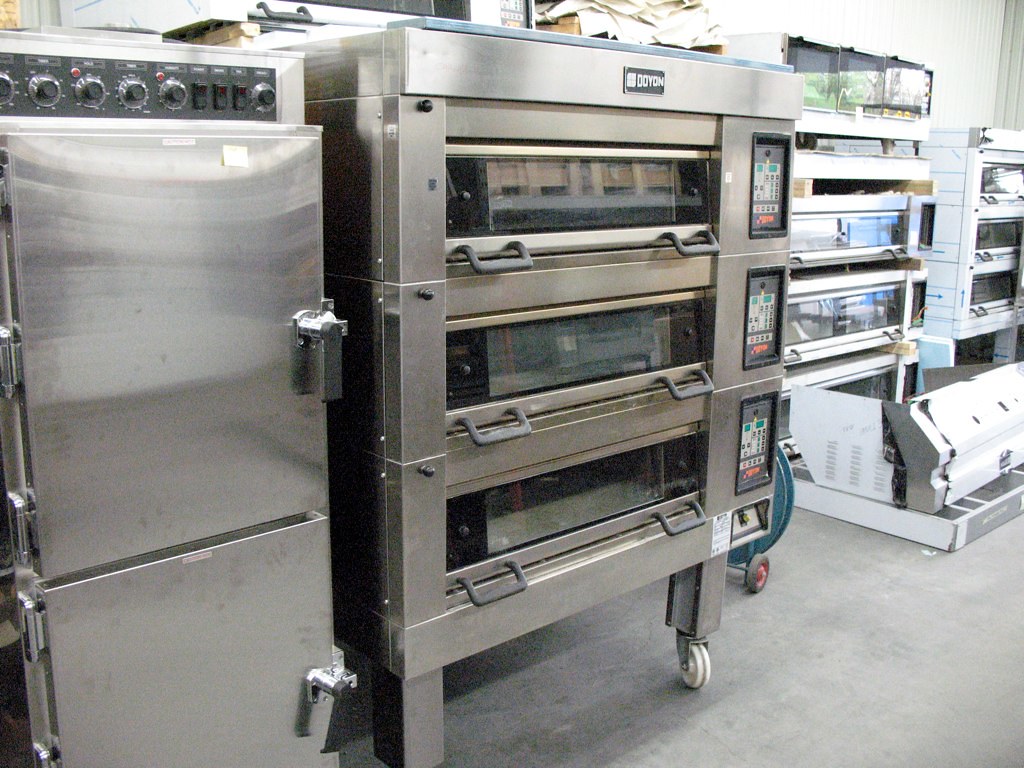This color photograph captures an industrial kitchen, possibly in a commercial restaurant or bakery, illuminated by bright sunlight streaming through a window or open door. The central focus is a stainless steel Doyon convection oven with three horizontally-aligned compartments, each featuring glass windows and dual silver-gray handles. This oven rests on wheels and is flanked by black touch panels adorned with blue, red, and white details.

To the left stands a tall, stainless steel piece of equipment resembling a refrigerator or freezer. It has two compartments, each with substantial handles, and a black rectangular panel on top equipped with six knobs and three flip switches.

In the blurred background to the right, additional stainless steel ovens and shelving units are visible. One of these background units also has a touch panel with buttons and lights. On the floor, there's another piece of unspecified machinery. The overall aesthetic is dominated by the gleam of metal surfaces, brightly highlighted by the sun, underscoring the robust, industrial nature of the kitchen.